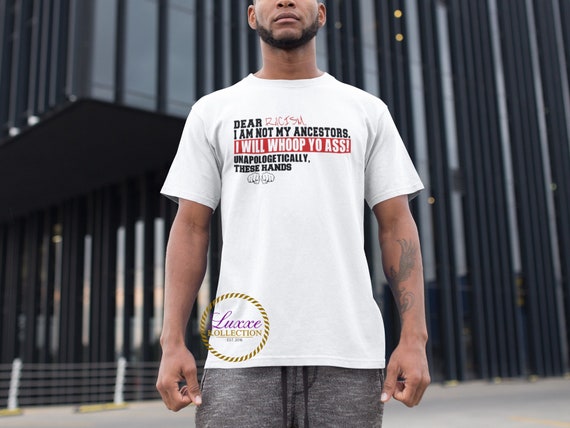The image features an African man, cropped from below his eyes down to his thighs, standing in front of a tall building with distinct black metal beams and glass panes. The lower part of the building's facade includes a small fence. The man has a trimmed black beard without a mustache and displays a large tattoo, possibly a phoenix, on his left forearm. He is dressed in a white, short-sleeved t-shirt with the following bold statement: "Dear Racism, I am NOT my ancestors. I will whoop your ass unapologetically. These hands," with the word "Racism" written in red handwritten font and the phrase "I will whoop your ass" in white font on a red banner, accompanied by illustrations of two fists. The shirt also features a small circle with the text "Luxxe Collection" and a gold border on the lower right side. He pairs this shirt with gray sweatpants with a visible dangling string.